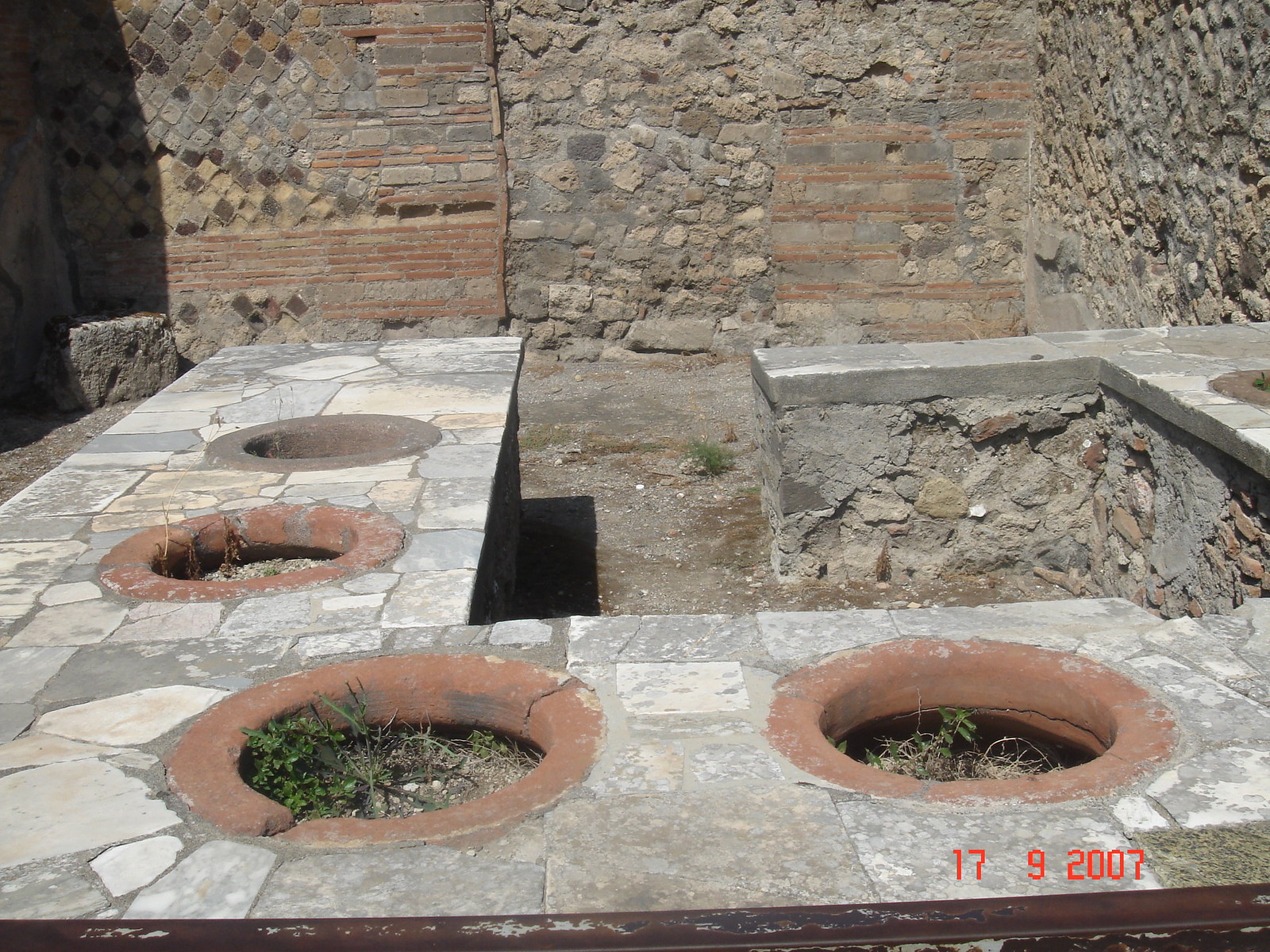This outdoor scene captures a fascinating mix of masonry and nature, set against a diverse background of bricks and stones, forming various patterns. The backdrop features a blend of red bricks, gray stones, and beige and tan hues that create stripes and random rocky formations. Central to the image is a raised seating area or patio base, approximately thigh-high, crafted from stones with a flat seating surface on top. Intriguingly, this structure includes four built-in flower pots made of red clay, positioned along one side, containing soil and weeds. Little patches of green grass peek through the stone flooring, adding a touch of nature to the predominantly stony environment. The photograph, dated September 17, 2007, conveys a sense of ancient architecture, reminiscent of historic brick and stone constructions.